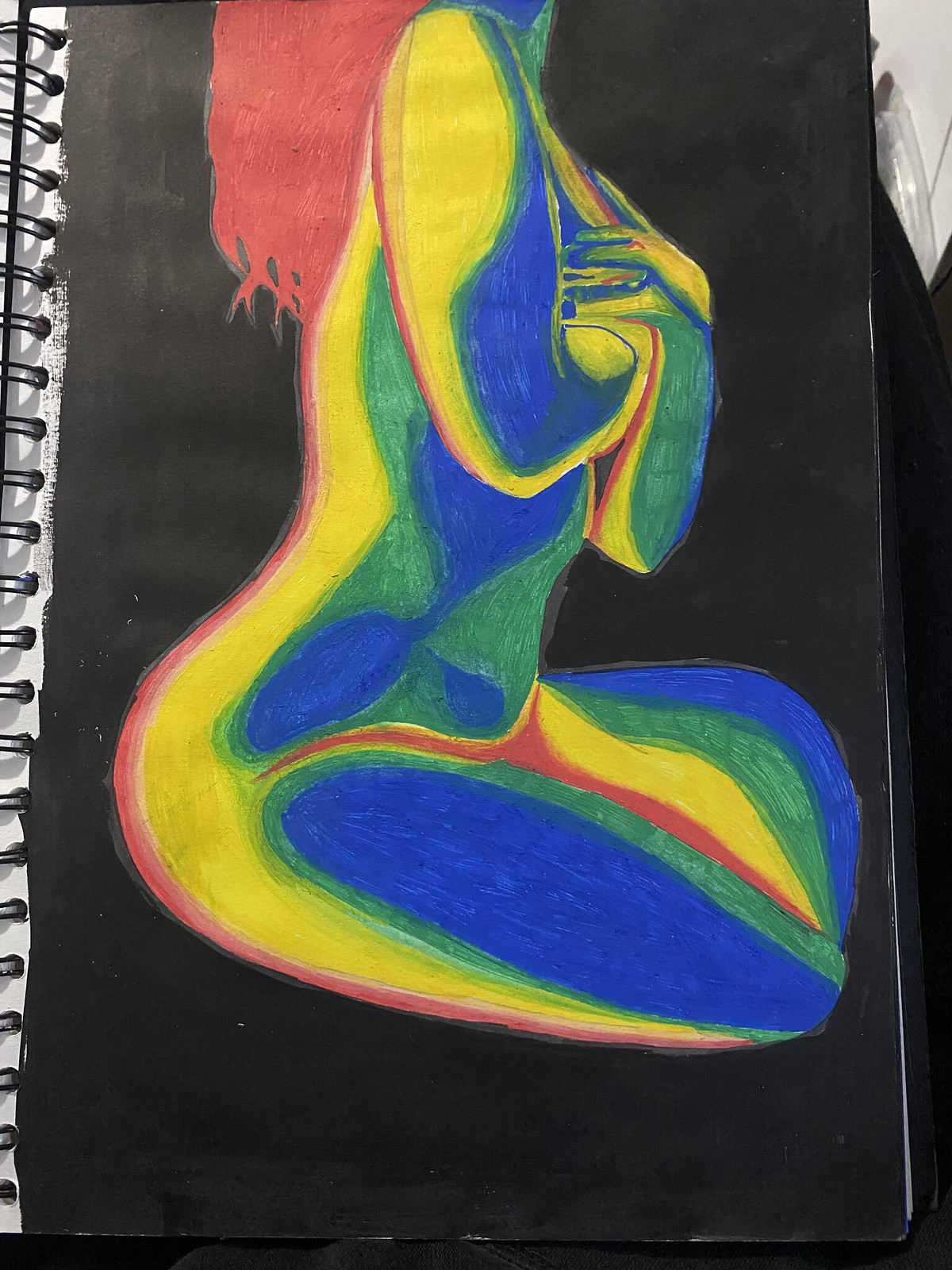This vibrant, color sketch captures the side profile of a young woman seated with her legs crossed and arms folded close to her chest. Rendered possibly with a mix of colored markers, pencils, or paint, the artwork is a kaleidoscope of hues. The girl's long, flowing orange hair cascades down her back, contrasting vividly with her body, which is an intricate mosaic of yellow, blue, green, and orange patches. The stark black background amplifies the colorful explosion, showcasing the woman's serene posture and contemplative expression in a striking, artistic manner.